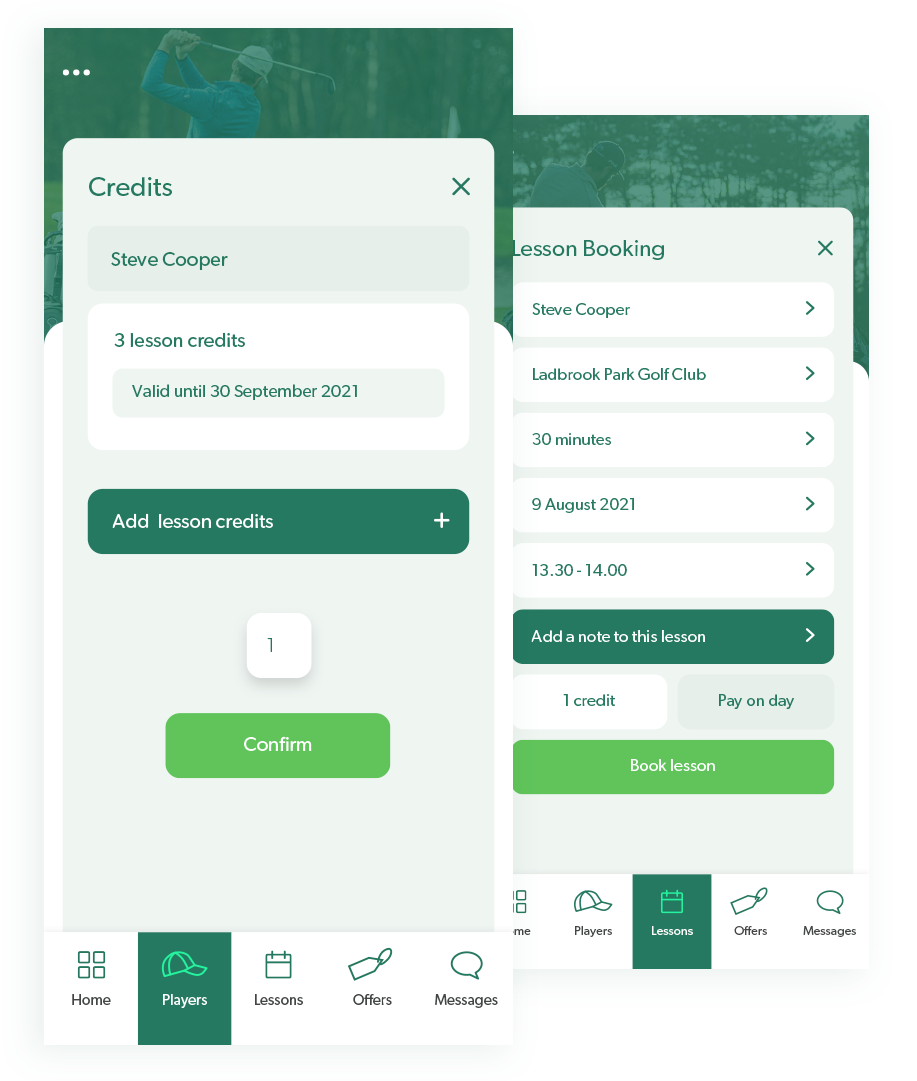These are two screenshots of the app. The left screenshot is larger and shows various elements of the app interface. At the top, there are three white dots followed by a photo of a golfer viewed from the back, holding up a golf club. The golfer is wearing a white hat and a blue shirt, and the image has a green filter overlay. 

Beneath this image, there's a white box labeled "Credits" with an "X" to the right. Below that is a grey box that says "Steve Cooper." Further down, there's another white box indicating "Three lesson credits." Below this, there's a green box labeled "Add lesson credit" featuring a "+" symbol. Beneath that is a white square with the number "1" inside it. Following that, there's a light green button labeled "Confirm."

At the bottom of this screenshot are five navigation buttons:
1. Four green squares labeled "Home."
2. A baseball cap labeled "Players," which is highlighted in green.
3. A calendar icon labeled "Lessons."
4. A tag icon labeled "Offers."
5. A speech bubble icon labeled "Messages."

Adjacent to the larger screenshot is a smaller one. Here, there is a button labeled "Lesson Booking," below which there are several elements:
- An arrow pointing to "Steve Cooper."
- An arrow pointing to "Ladbroke Park Golf Club."
- An arrow pointing to "Thirty minutes."
- An arrow pointing to "9 August 2021."
- An arrow pointing to "13:30 to 14:00."
- A green button labeled "Add a note to this lesson" with an arrow.

Lastly, below these elements, there's text indicating "One credit" next to "Pay on day," and beneath that, a green button labeled "Book lesson."